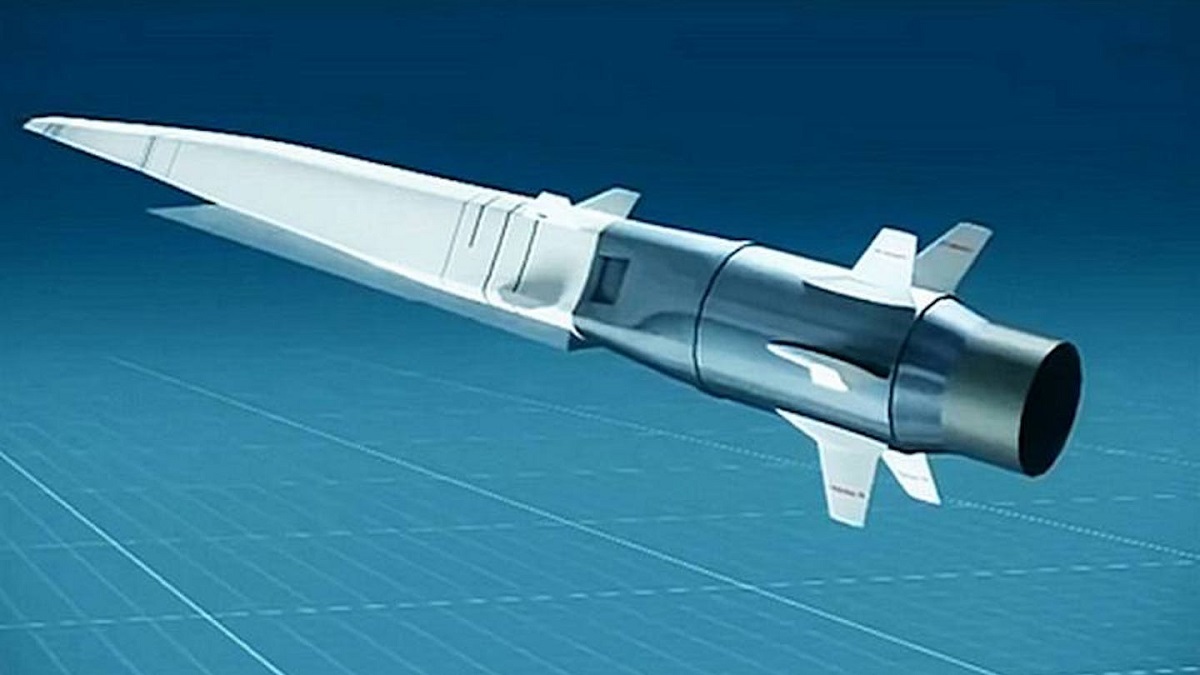In the image, a futuristic and mechanical object is set against a striking blue ombre background which transitions from dark blue at the top to a lighter blue at the bottom, featuring grid-like lines. The central object, resembling a knife or a missile, has a sharply pointed white tip on the left and a darker blue or black handle-like end on the right. This object, possibly a 3D computer mock-up, is adorned with various protruding elements suggesting it has functional parts. The detailed background and floating presentation of the object give it an advanced, almost sci-fi feel, akin to design aesthetics seen in films like Tron. The object's white tip contrasts starkly with the darker, possibly twistable end, emphasizing its sleek and innovative design.